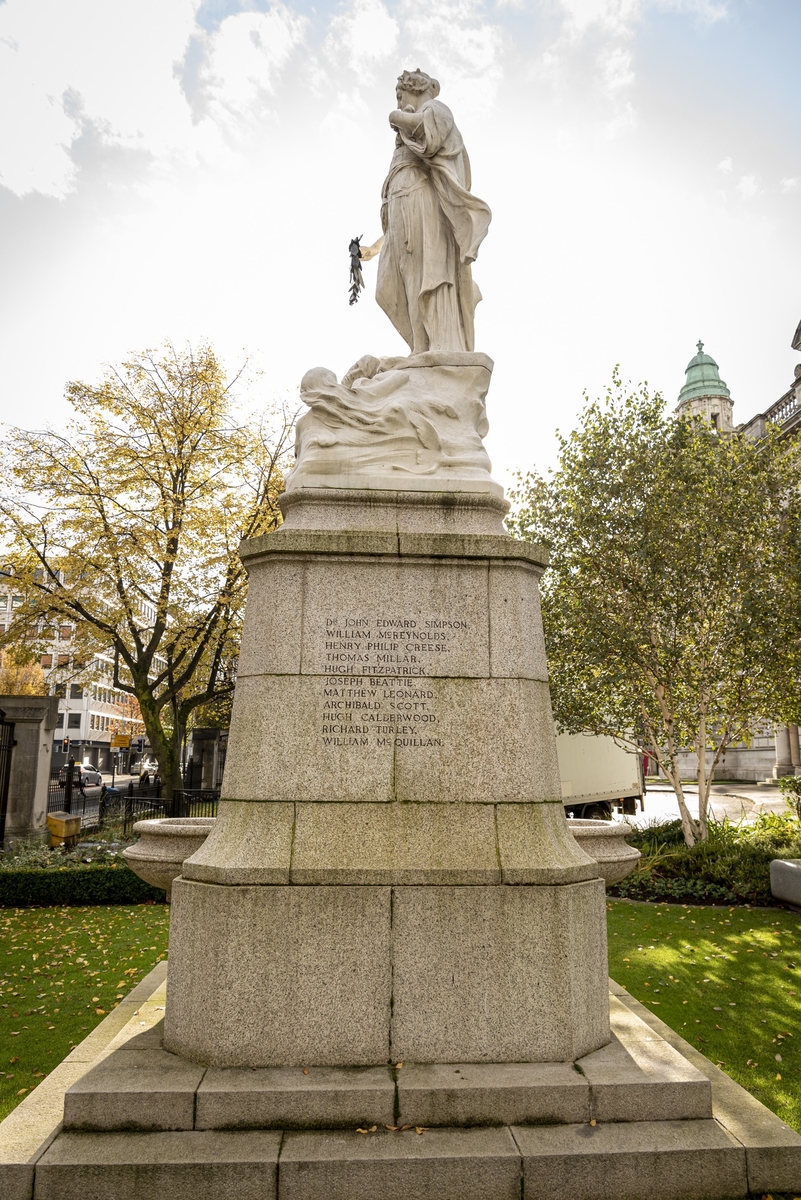The image features a striking statue situated in a park-like courtyard, observed from a side angle. The statue, made of what appears to be granite or marble, stands upon a tall white pillar. It depicts a woman in classical or Grecian attire, holding a branch or plant in her right hand, with her left arm bent gracefully towards her mouth. The base of the statue is inscribed with several names, likely to be benefactors or individuals commemorated by the statue. The statue shows signs of mildew and age, resting on green grass with leaves scattered around. In the background, the scene is set on a partly cloudy day, with bright blue sky peeking through the clouds. Surrounding the statue are trees and several older-looking buildings, including a possible capitol building, indicating a downtown city area. Additionally, a truck and some distant cars are visible, further situating the statue within an urban environment.